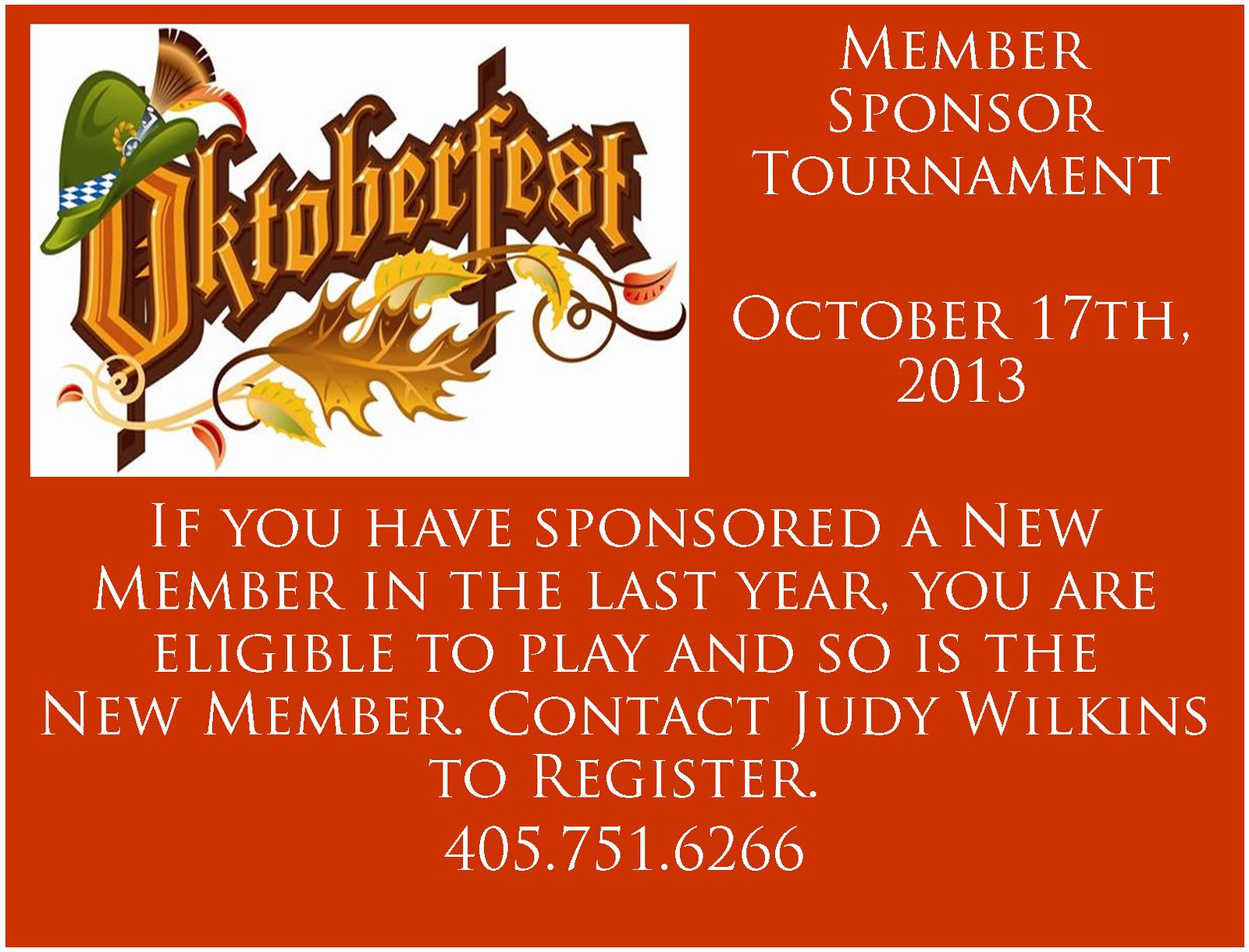This poster is an eye-catching, festive advertisement for an Oktoberfest Member-Sponsored Tournament, taking place on October 17, 2013. The background of the poster is a vibrant red, with large and stylish white lettering that is designed to immediately grab your attention. Prominently featured on the left side is the word "Oktoberfest" in yellow letters within a white background rectangle, with colorful fall leaves adorning the bottom. A whimsical green hat with a feather is perched on the "O" in "Oktoberfest," enhancing the festive feel of the design. Below the announcement, it's detailed that if you have sponsored a new member in the past year, both you and the new member are eligible to participate in the tournament. To register, contact Judy Wilkins at 405-751-6266. Overall, the poster’s striking colors, creative fonts, and playful imagery make it both visually appealing and informative.